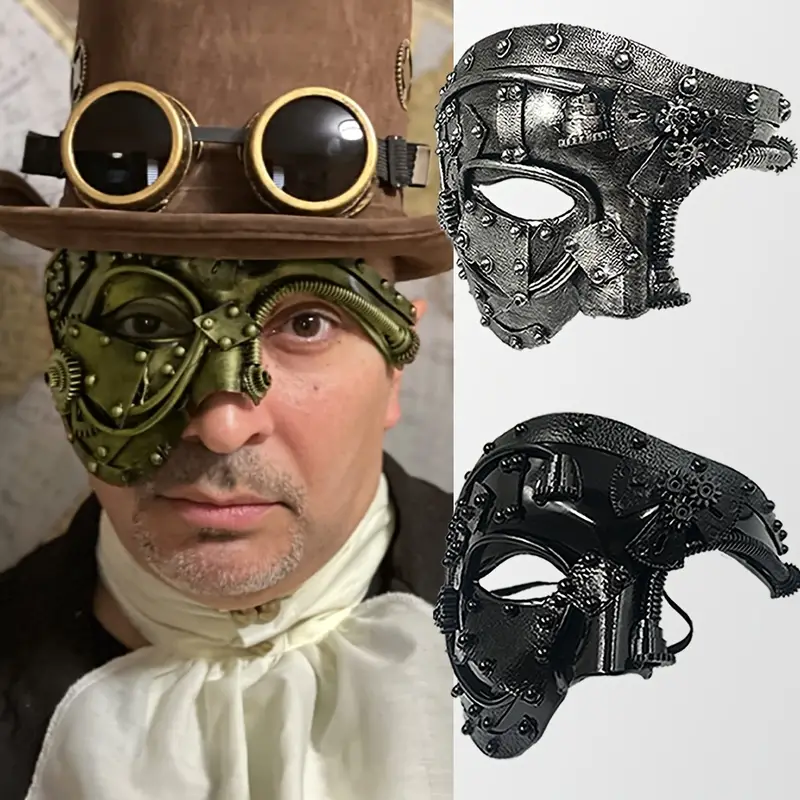The image is vertically divided into two sections, with the left side being larger. On the left, we see a man adorned in a black top hat, which has black goggles with yellow trim resting on its brim. The man wears a steampunk-inspired greenish metal eyepiece that covers one eye and extends over the other, though it remains uncovered. This elaborate device includes screws, sprockets, and small metal balls, giving it a distinctive mechanical look. He has a light beard and mustache, and stares directly into the camera without smiling. His attire consists of an old-fashioned black coat over a white billowed-out shirt, fastened at the neck with a goldish button or clasp. On the right side of the image, set against a gray background, are two other eyepieces similar to the one he is wearing. One is silver, with designs akin to his, and the other is black, featuring round sprocket details and small attached balls. These additional masks appear to be alternative versions available for purchase.